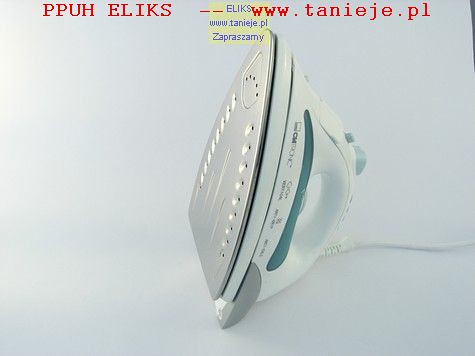This image is an advertisement for a white, steam iron with a white and aquamarine blue design, prominently displayed against a grayish-white background. At the top of the photo, there's red text in another language, likely Polish, which reads "P-P-U-H-E-L-I-K-S," followed by the website "www.tanieje.pl." The iron is shown standing upright, with a visible chrome surface and detailed steam jets on its base. It also has a clear water level bubble and several buttons on top. The cord extends out to the right and there's tiny, indiscernible writing in gray near the base. The background is minimalistic, with no identifiable setting, making the iron the focal point of this well-lit and clean advertisement.